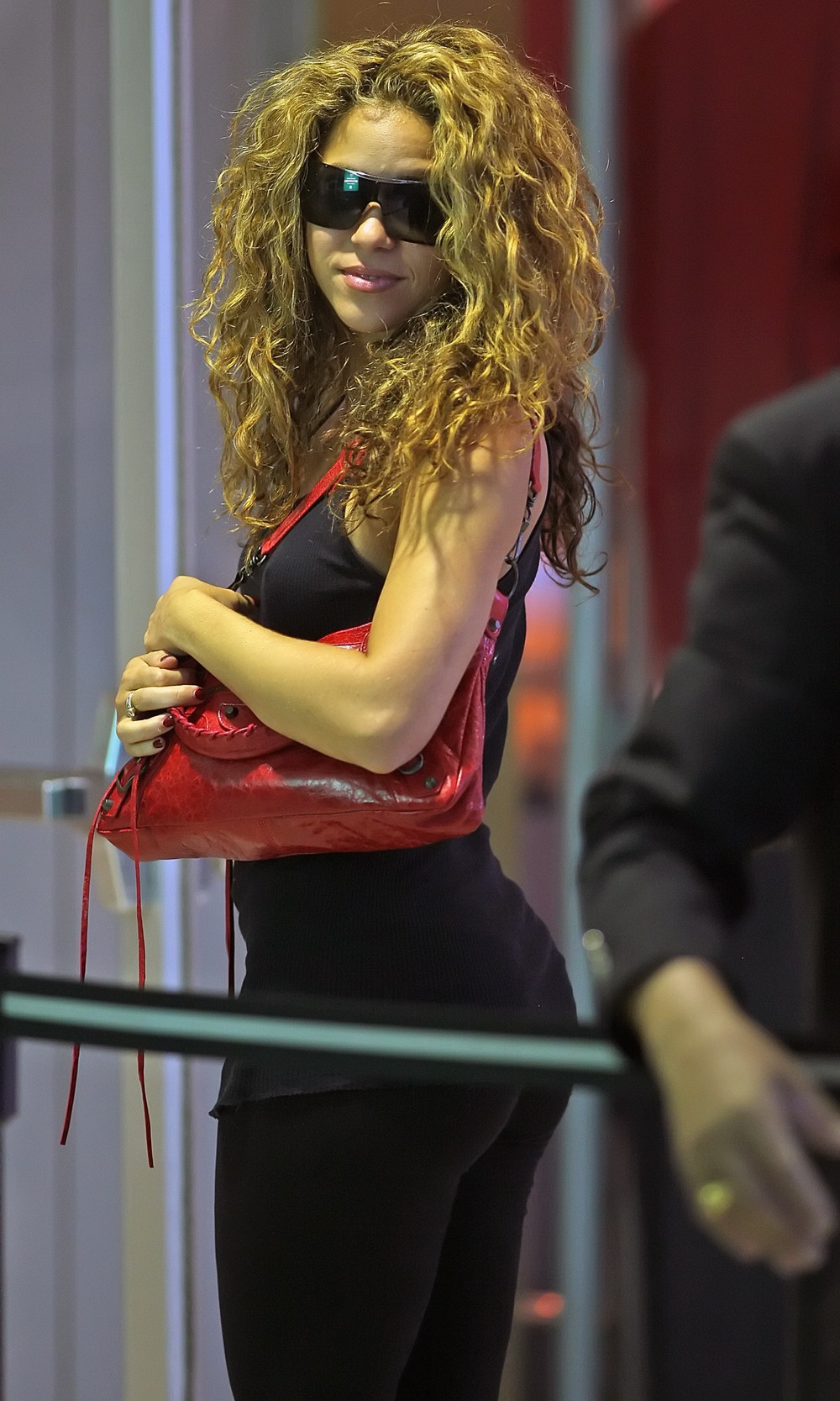The image features a woman who closely resembles singer Shakira, but due to her large sunglasses, it's hard to confirm if it is indeed her. She has long, wavy, and fluffy blonde hair. She's wearing a black tank top and black leggings, and she carries a large red purse on her left shoulder, holding onto the straps with both hands. Her nails are painted red. The woman is facing left, but her head is turned forward, looking toward the front of the image. In the background, there are blurry white and red curtains. To the right, a man's shoulder and arm, which appears to be wearing a black suit jacket, suggest the presence of security. There's also a black and white barrier ribbon cutting across the image, adding a sense of division.